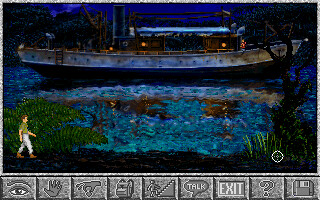The image features a series of gray icons aligned at the bottom. From left to right, the icons include an eye, a hand symbol, a hand pinching something, an iPad, and an icon of people walking up stairs. This is followed by a speech bubble with the word "talk" inside, an icon representing exercise, a question mark, and a floppy disk. 

To the left of this sequence stands a person in a green shirt, blue pants, and with short brown hair. Surrounding the person on both sides are lush green leaves. In the center of the image, a metal boat is depicted, with a part resembling a blue-topped steamboat visible.